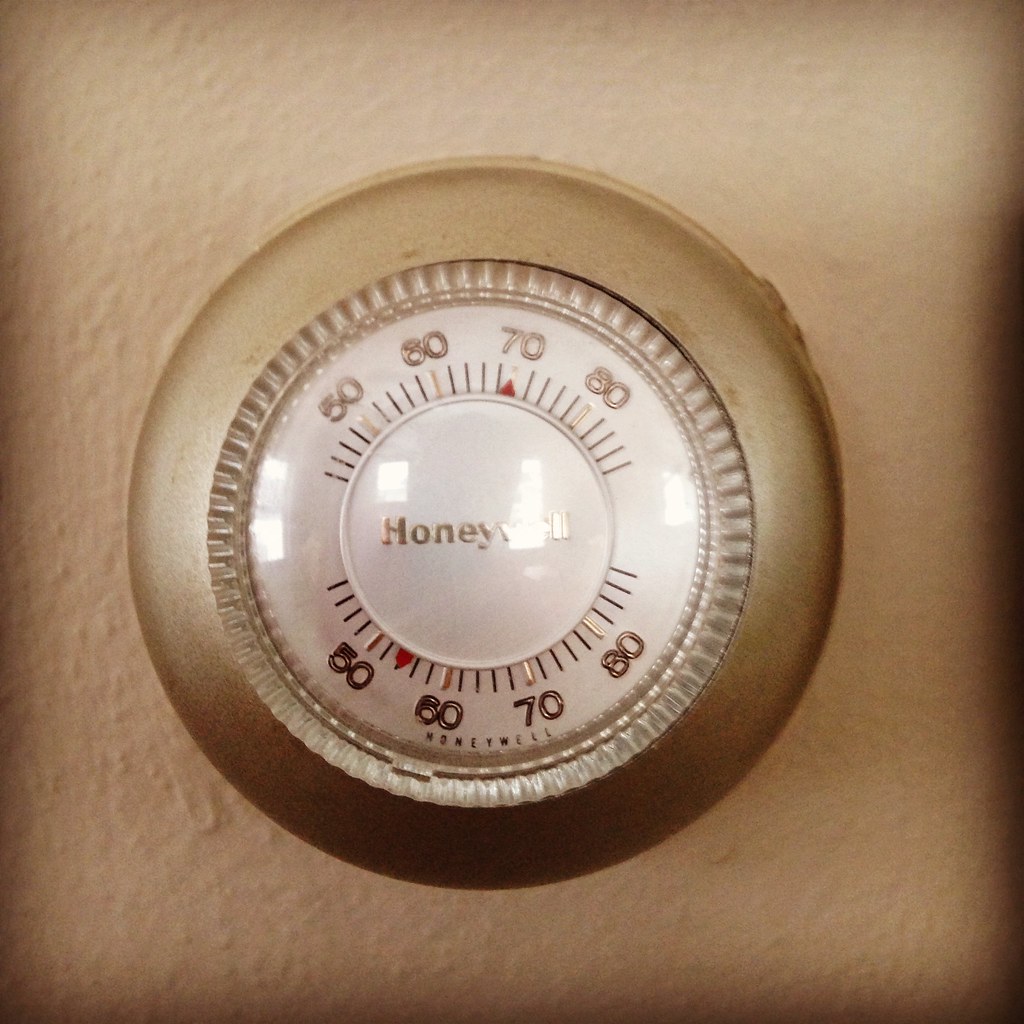This vintage photograph captures an old-school Honeywell thermostat mounted on a wall that appears almost gold due to the yellowish filter applied, giving the image an antiquated feel. The thermostat features a metallic gold bezel encircling a transparent, twistable knob used to adjust the temperature setting. Centrally positioned on the device is a white circular display with finely marked temperature lines ranging from 45 to 85 degrees. Gold letters spell out the Honeywell brand name at the center of this display. The thermostat intriguingly showcases two sets of temperature lines, likely for separate heating and cooling settings. In this particular scene, the top gauge is set to 70 degrees, while the bottom gauge is set to 55 degrees, highlighting the distinct historical charm and technological approach of this bygone temperature control device.